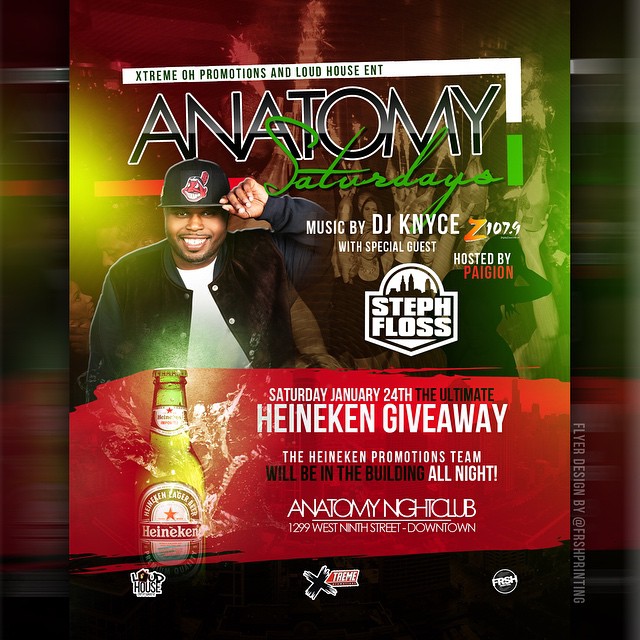The poster is a vibrant, promotional advertisement for "Anatomy Saturdays" at the Anatomy Nightclub, located at 1299 West 9th Street, Downtown. Dominating the top of the poster is the bold title "Anatomy Saturdays," with "Anatomy" in black capital letters outlined in white, and "Saturdays" in a bright green cursive font. The event features music by DJ KNYCE (DJ Nice), with a special guest appearance by Steph Floss, hosted by Pagion, whose name is prominently displayed in white text and red small letters. 

An image of a black gentleman, likely a rapper, graces the left side of the poster. He is seen wearing a black jacket and a black Chiefs baseball cap with a red logo, along with a white t-shirt underneath. He poses with a smile, his hand holding the rim of his cap.

The main text of the poster, written in white, announces "Saturday, January 24th, the Ultimate Heineken Giveaway," with details stating that the Heineken promotion team will be present all night. To the left of this text is an image of a Heineken bottle, cap still on, adding to the enticing promotional allure.

Noteworthy logos for Extreme OH Promotions and Loud House Entertainment are visible, with the Loud House logo being part of the event branding. There's a red tint background which subtly depicts what appears to be marijuana buds, softened by color filters.

At the bottom right corner, the poster credits the design to FRSH Printing in a vertical orientation. Overall, this detailed promotional flyer, with its striking mix of images, text, and branding elements, effectively captures the essence of a lively night at the Anatomy Nightclub.